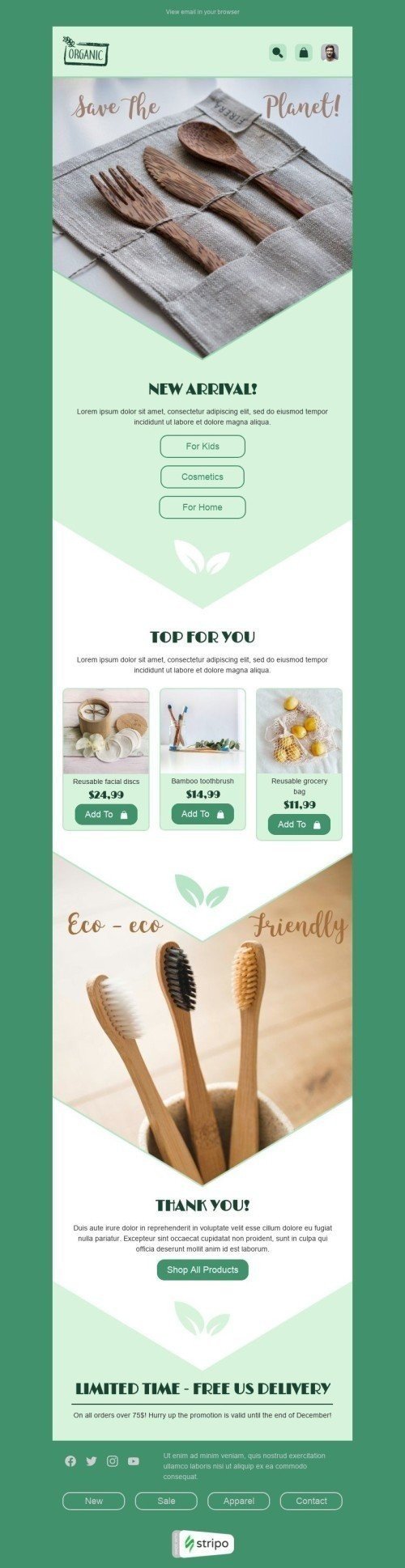The image is a vertically aligned rectangle with a thick green border. At the top, it features the text "Save the Planet" against a light green background. Below this text is a cloth napkin made of tan-colored fabric, containing a wooden fork, knife, and spoon. The middle of the image includes the phrase "New Arrivals" in green text, though the rest of the accompanying text is too small to read. Midway down, the background shifts to white with the text "TOP FOR YOU" in all caps in green. Beneath this, there are three vertical images with prices, although the details are also too small to read.

Near the bottom, the background changes to a wood counter, displaying the words "eco-friendly" and a cup with three wooden toothbrushes sticking out. The image is part of an online ad from a company called Stripo, known for offering eco-friendly items like organic wooden utensils, reusable facial disks, bamboo toothbrushes, and reusable grocery bags. Additionally, there are buttons and text interspersed, including a section with a Latin placeholder phrase and a call to action for U.S. customers about free delivery for a limited time.